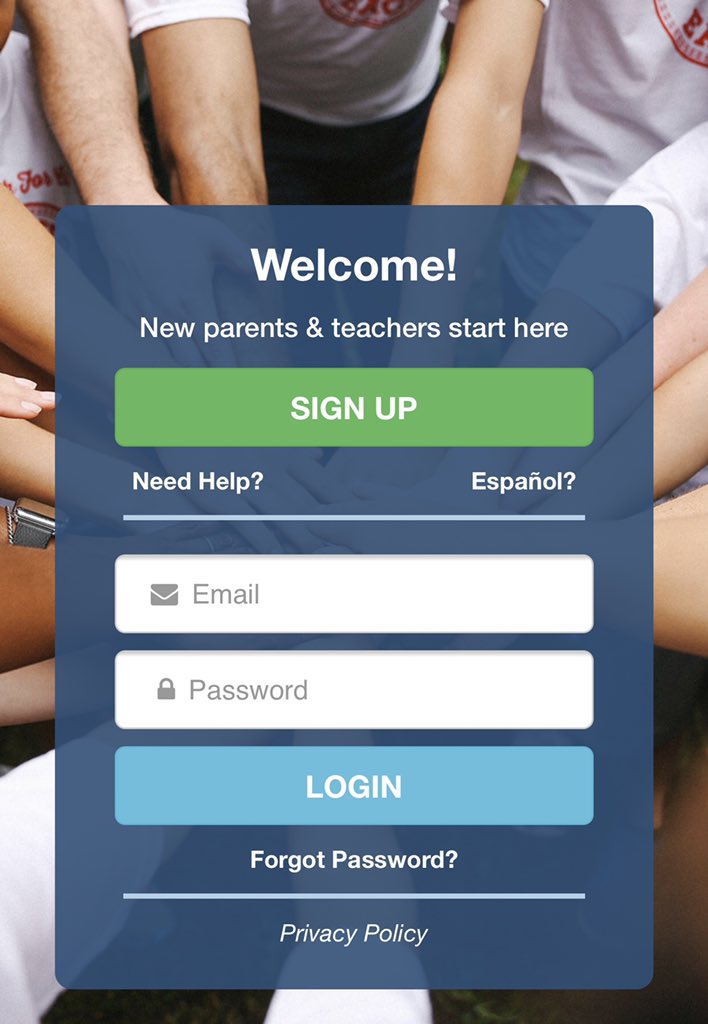The image features a blue background with a prominent central message in bold white text stating "Welcome!" Beneath this, slightly smaller in bold white text, it reads "New Parents and Teachers Start Here." A green tab spans the width of the image, displaying "Sign Up" in white text.

Surrounding the central text, multiple arms extend towards the middle from various directions—top, right, and left. The individuals are wearing short-sleeve white t-shirts, and only their forearms are visible. No hands are visible at the bottom due to a blue pop-up tab.

In the bottom left corner, next to the green "Sign Up" tab, the text reads "Need Help?" while the right side says "Español?" Both are marked with a question mark and separated by a thin blue line. Below this line is a white rectangle with an email icon and the word "Email" in black. Below it is another white rectangle featuring a lock icon and the word "Password."

At the very bottom, another blue tab stretches across the image, displaying "LOGIN" in white, all capitals. Underneath, there is smaller white text stating "Forgot Password?" followed by another thin blue line and the text "Privacy Policy" in white at the very end.